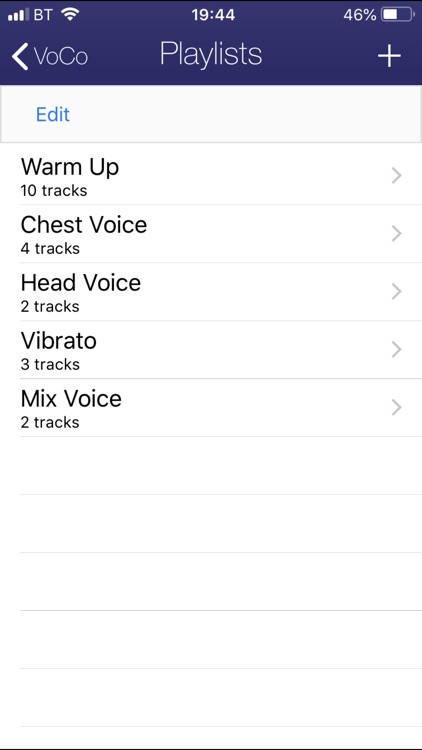The screenshot is captured from a smartphone, showcasing the following details:

At the top, there is a navy blue border that houses several icons. On the right side of this border, a white battery icon indicates that the battery is 46% charged. In the center, the time is displayed as 19:44, indicating the 24-hour clock format. The left corner shows "BT," followed by signal bars representing the wireless connection, with three out of four bars filled. To the right of this, the Wi-Fi icon is visible.

Beneath this top section, in thin white font, there is the word "Playlist" in the middle. On the left side, underneath "Playlist," the label “the VOCO” is displayed, where "V" and "C" are capitalized, and an arrow pointing to the left is on the left of this text. On the right side, opposite of "the VOCO," there is a white plus sign.

The main portion of the screen is white, embedded with a list of tracks. At the top-left corner, "Edit" is written in blue font. Below this, the list of tracks is presented in dark gray font. The first item is "Warm Up," which has 10 tracks indicated by the text "10 tracks" beneath it. To the right of "Warm Up," there is an arrow suggesting a drop-down menu for track details. The subsequent items are:

- "Chest Voice" with 4 tracks
- "Head Voice" with 2 tracks
- "Vibrato" with 3 tracks
- "Mixed Voice" with 2 tracks

Each item follows the same format, with the number of tracks listed beneath the track name and a right-facing arrow on the right side.

At the very bottom of the screen, a very thin black line is visible, marking the end of the list.

This detailed screenshot offers insight into the organization and user interface of a playlist feature on the smartphone.